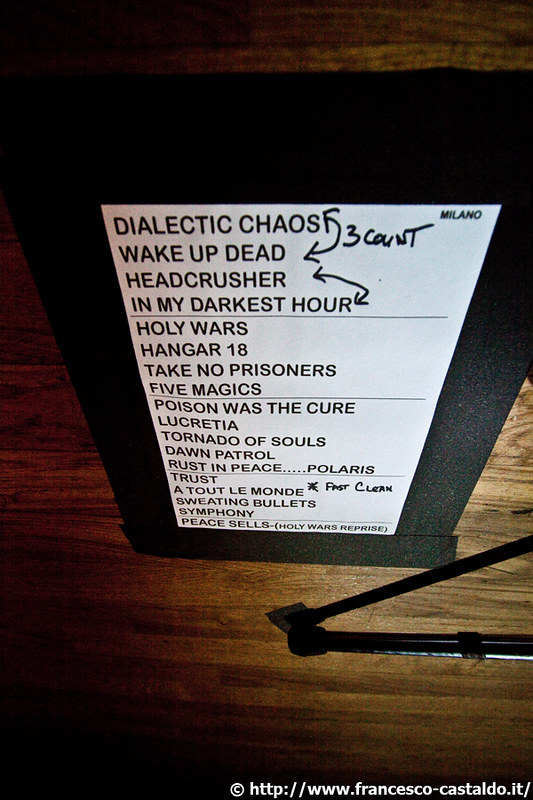The photograph showcases a detailed label positioned either on a wooden table or wall, with the background featuring horizontal slats of brown wood, darkened in the upper left and lower left corners. Central to the image is a shiny black rectangular object displaying a white paper section with black text. A watermark bearing the copyright symbol and URL "http://www.francesco-castaldo.it/" appears in the lower right corner. 

The white paper lists numerous phrases and song titles in bold black print, organized into distinct sections separated by horizontal lines. The first segment reads "dialectic chaos, wake up dead," with a hand-drawn connecting arrow and the handwritten note "three count" beside it. The next lines are "headcrusher" and "in my darkest hour," connected by another arrow. 

The second section includes "holy wars, hangar 18, take no prisoners, five magics." Following a pinstripe separator, the third section lists "poison was the cure, Lucretia, tornado of souls, dawn patrol, rust in peace - Polaris," with another pinstripe below it. The final section reads "trust, a tout le monde, sweating bullets, symphony," with an asterisk beside "a tout le monde" and the note "fast clean" written by hand. The list concludes with "peace cells (holy wars reprise)."

In the upper right corner of the white paper, the word "Milano" is printed. The intricate details combined create a meticulously organized and annotated list on a rustic wooden backdrop.